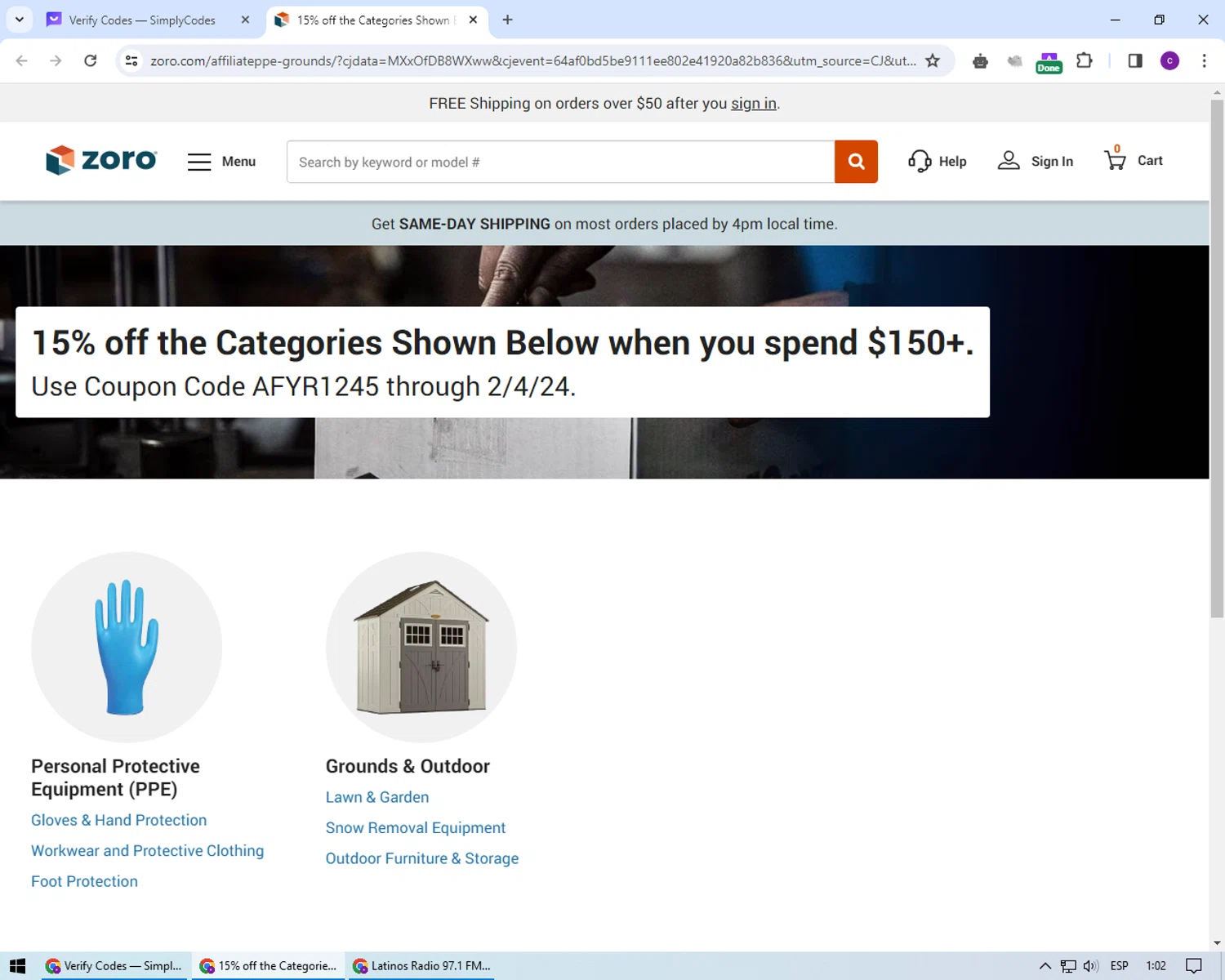Screenshot of the Zorro.com website home page, showing two tabs open in the browser. The active tab is dedicated to code verification, titled "Verify Codes." The website features a prominent gray banner at the top, which reads "Free shipping on orders over $50 after you sign in." The Zorro logo is displayed prominently, adjacent to a navigation menu offering options to "search by keyword or model number," seek "help," "sign in," and view the "cart."

Below the navigation menu, a notification reads "Get same day shipping on most orders placed by 4 p.m. local time." Another promotional banner follows, stating "15% off the category shown below when you spend $150 or more. Use coupon code AFYR1245 through February 4th, 2024."

The website's main content includes a category list starting with PPE (Personal Protective Equipment), represented by an image of a glove. Beneath this section, detailed subcategories are listed: "Gloves and Hand Protection," "Work Wear and Protective Clothing," and "Foot Protection," indicating a comprehensive range of body protection gear. Adjacent to the PPE category is the "Grounds and Indoor" category, offering items such as "Lawn and Garden," "Snow Removal Equipment," and "Outdoor Furniture and Storage," along with an image of a small shed.